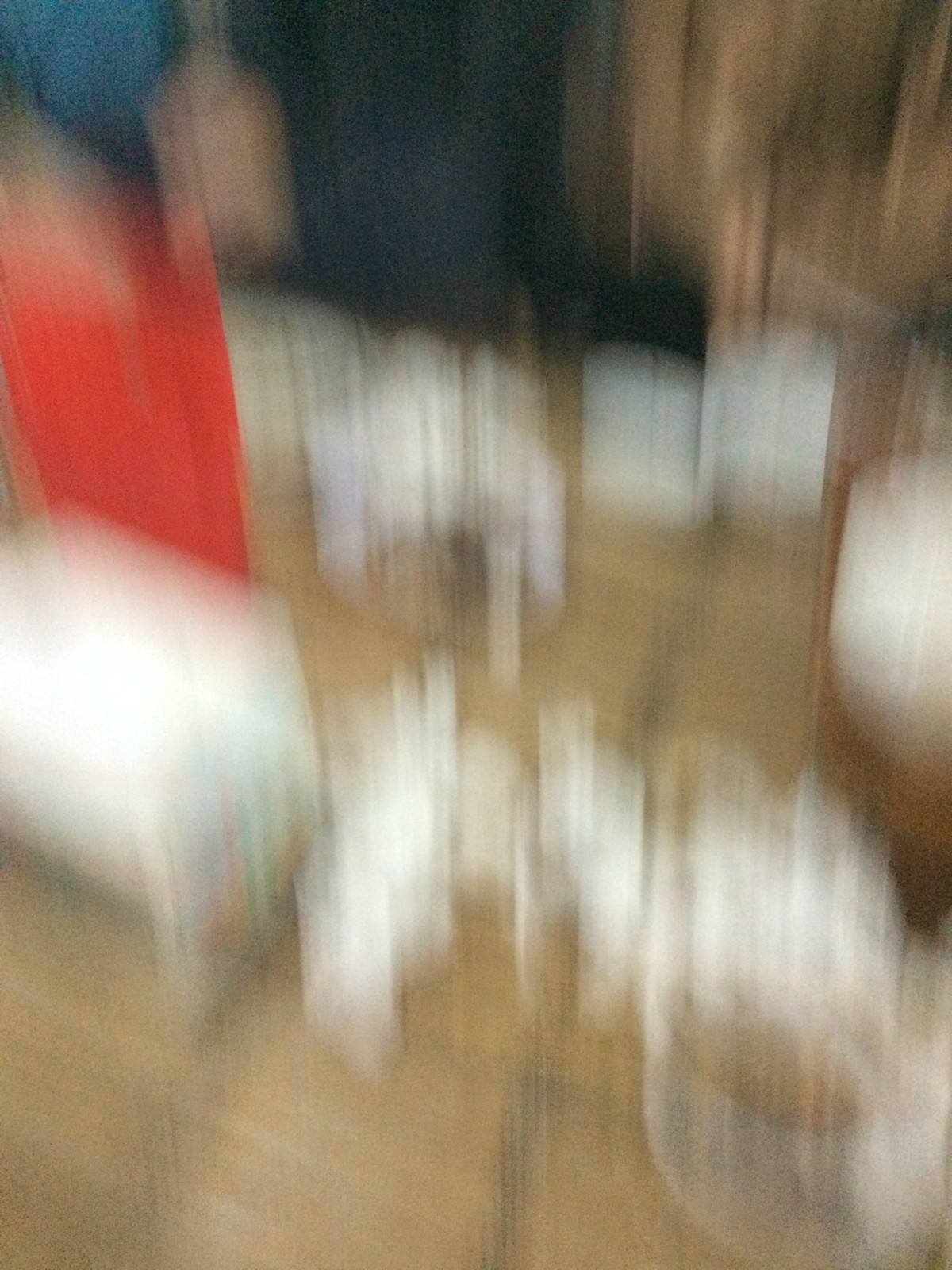In this photograph, significant vertical motion blur obscures the scene, making it challenging to discern specific objects and details. The image is dominated by streaks of red, brown, white, and blue colors, all extending vertically due to the camera shake. The brown tones suggest a wooden table, possibly in a restaurant setting. On the left side, the white areas likely indicate napkins arranged with various glassware, including a notable red-colored glass. The blue streaks probably represent a person wearing a blue shirt, while the tan hue on one side might be an arm. Despite the overall indistinctness, these colorful blurs hint at a casual dining environment.